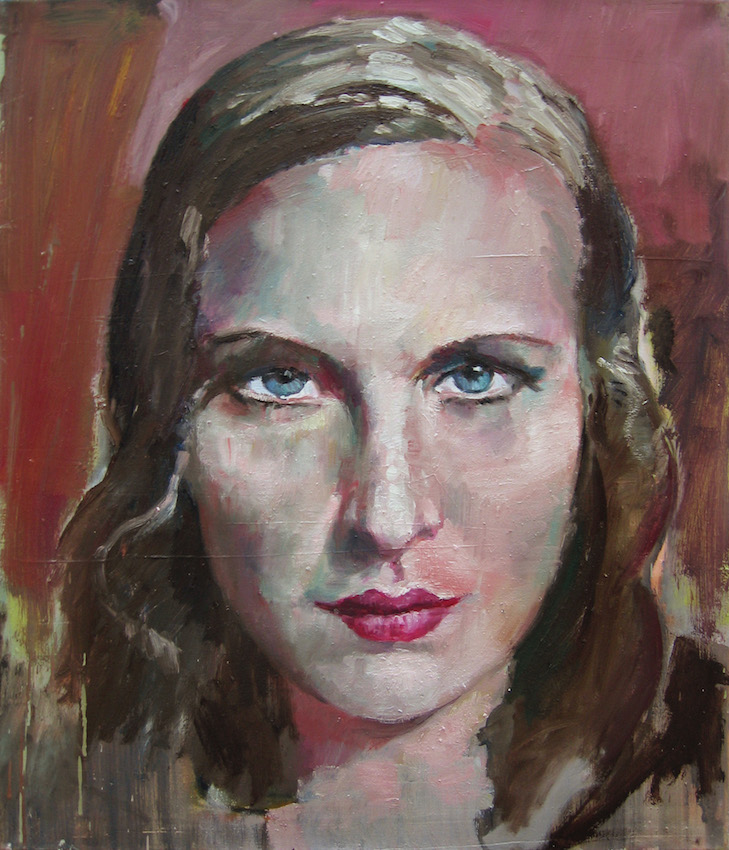In this watercolor painting, a woman with stark blue eyes and shoulder-length, light to medium brown hair stares directly ahead with a stern, focused expression. She has a pale complexion highlighted by blush tones that accentuate the shadows on her face and under her neck. Her thin eyebrows subtly define the shape of her eyes, and her lips are brightly painted red. The portrait is framed just above her shoulders, revealing minimal parts of her neck and a brown or black garment draped over her shoulders. Behind her, the background features a maroon to pinkish-red gradient, with darker hues on the left and lighter, more pinkish tones on the right, providing a rich, textured contrast to her serious demeanor.